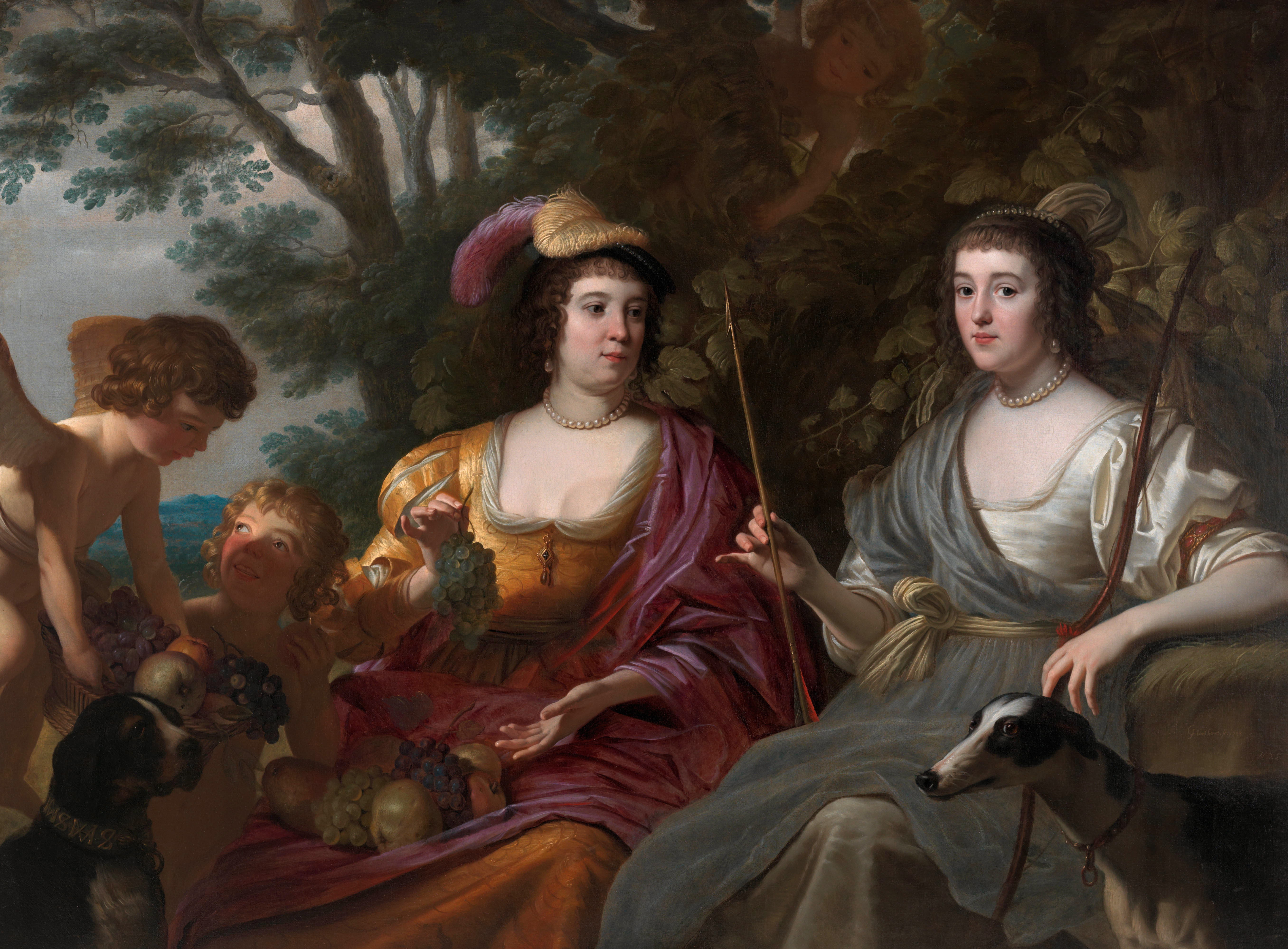The painting depicts an outdoor scene with two seated women surrounded by angelic figures and animals, evoking a serene, almost ethereal atmosphere. On the left, a woman with dark brown hair, adorned with a feathered hat and a pearl necklace, wears a gold and orange gown. She holds a cluster of white grapes in her right hand while an assortment of fruit, including pears, peaches, and grapes, rests on her lap. Beside her, another woman with similarly fair, pale skin and brunette hair, also wearing a pearl necklace, is dressed in a gray and white gown with a golden sash around her waist. At the woman's feet, a black and white greyhound-like dog stands attentively. To the left of the women, two cherubic figures, or toddlers with angel wings, each with curly hair—one brunette, the other blonde—bring a sense of whimsy and innocence to the scene. A tricolor spaniel dog sits near them, adding to the tranquil and pastoral setting. The background features lush, dark trees against a gray sky, rendering a soft, realistic texture that underscores the painting's detailed and harmonious composition.